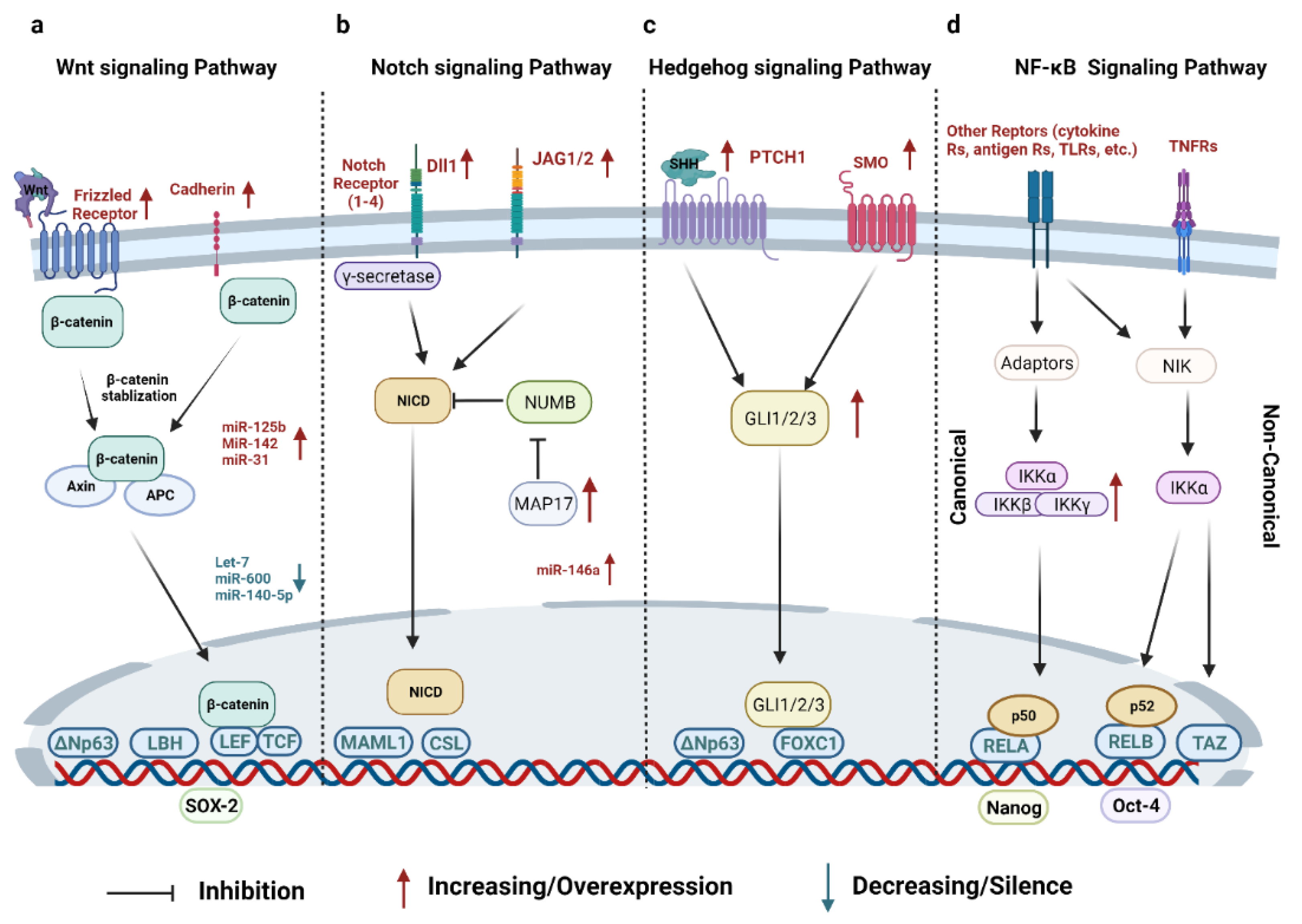This image is an informational diagram on a white background, divided into four vertical sections labeled A, B, C, and D. Each section details a different signaling pathway: WNT, Notch, Hedgehog, and NF-KB, respectively. Each pathway is depicted with various color-coded circles and illustrations:

- Section A (WNT signaling pathway) features black lowercase 'a' text and diagrams in green and blue.
- Section B (Notch signaling pathway) includes circles in purple, yellow, green, and blue with black text.
- Section C (Hedgehog signaling pathway) presents circles in yellow and blue with various icons.
- Section D (NF-KB signaling pathway) showcases circles in pink, off-white, purple, yellowy-orange, and blue.

A blue and purple curved line arches across the entirety of the diagram, connecting all sections, while additional colored lines and arrows indicate the flow and interaction within each pathway. At the bottom, a blue half-circle and a red-blue spiraled line highlight regulatory aspects. The bottom-most section includes a black line labeled "inhibition," a red arrow indicating "increasing overexpression," and a blue arrow for "decreasing silence."

Key elements mentioned across the pathways include receptors like frizzled receptor, counterin, notch receptor 1-4, D11, JAG1.5, PTCH1, SMO, and TNFRs. The last section also notes "canonical and non-canonical" pathways. Additionally, "October 4th" is indicated at the bottom of the diagram, possibly denoting a date or a reference point.